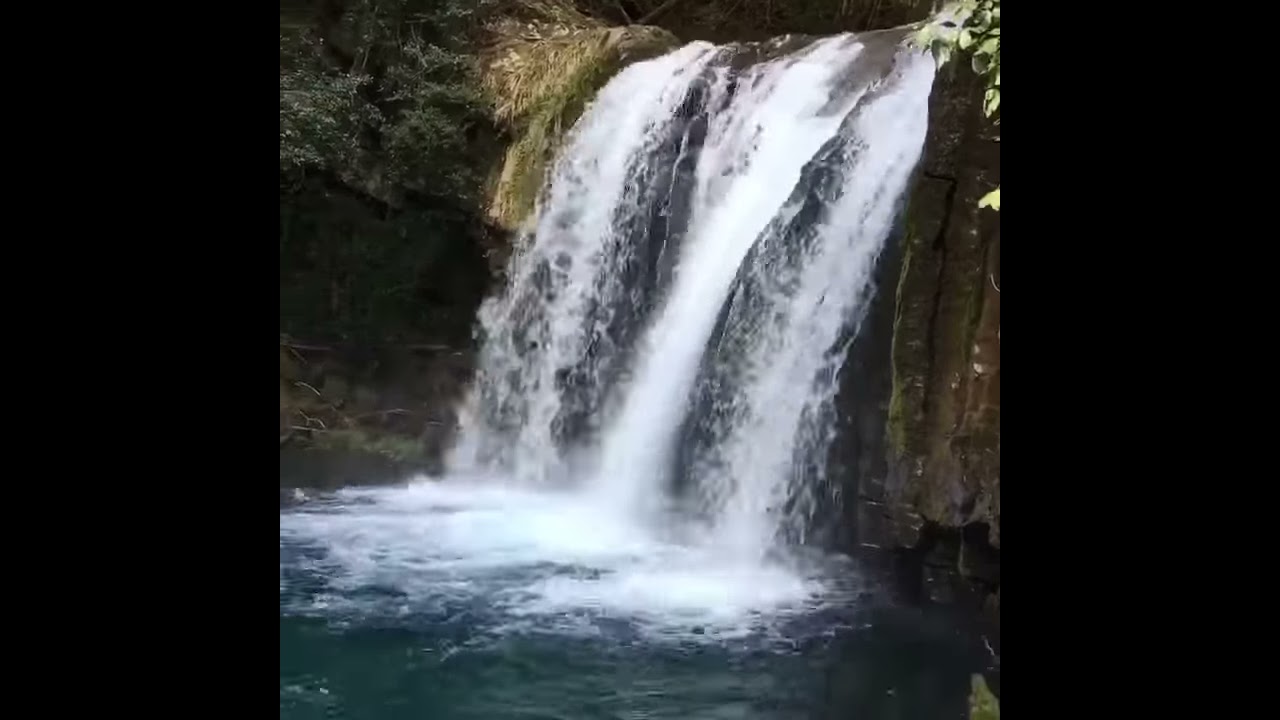The image showcases an impressive waterfall cascading from the upper right, plunging about 30 to 50 feet over a brown, granite cliff adorned with green vines and mold on its left side. The waterfall splits into three prominent, frothy white streams, rich with oxygen, creating a dramatic, misty spray as they hit the deep blue-green pool below. Set in what appears to be a lush, sunlit tropical forest, the surrounding foliage and illuminated trees in the background add to the serene, natural ambiance. The rocky cliff and vibrant water contrast beautifully, making this nature scene particularly captivating.